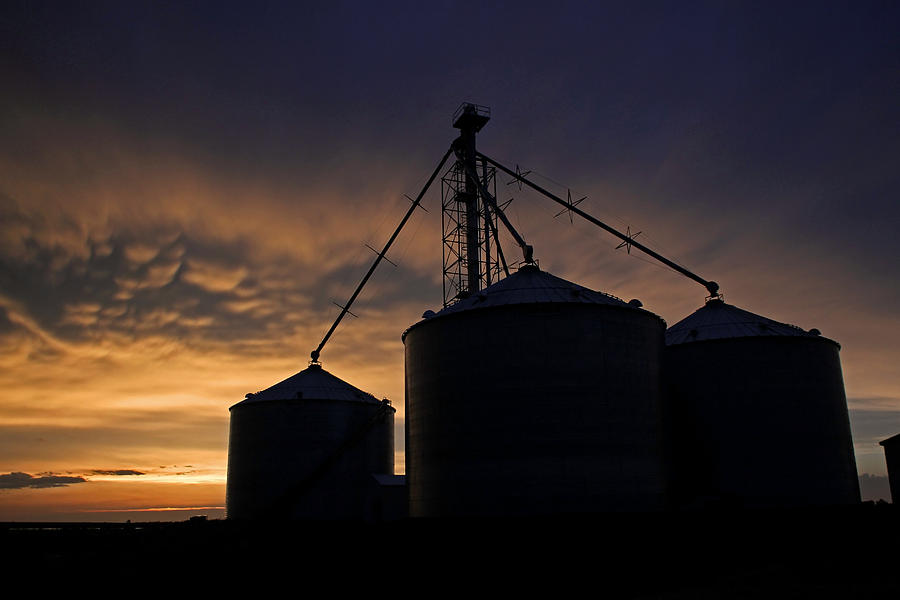The image captures an outdoor scene at sunset. The sky transitions from a bluish-gray in the upper part to orange and yellow hues where the sun is setting, creating a dramatic effect with the light filtering through the clouds. The right side of the sky features a deeper blue that fades into the scene's overall darker tones, surrounding vibrant orange and yellow clouds. Silhouetted against this vibrant backdrop, three green silos stand prominently. The largest silo appears more central, with the remaining two positioned slightly behind and to the side. These silos, connected by a network of poles and an elevated grid-style frame with a landing and handrails, cast striking shadows on the ground below. The ground level is a silhouette, with blurred mountain ranges visible in the distance, further enhancing the depth and composition of the image.